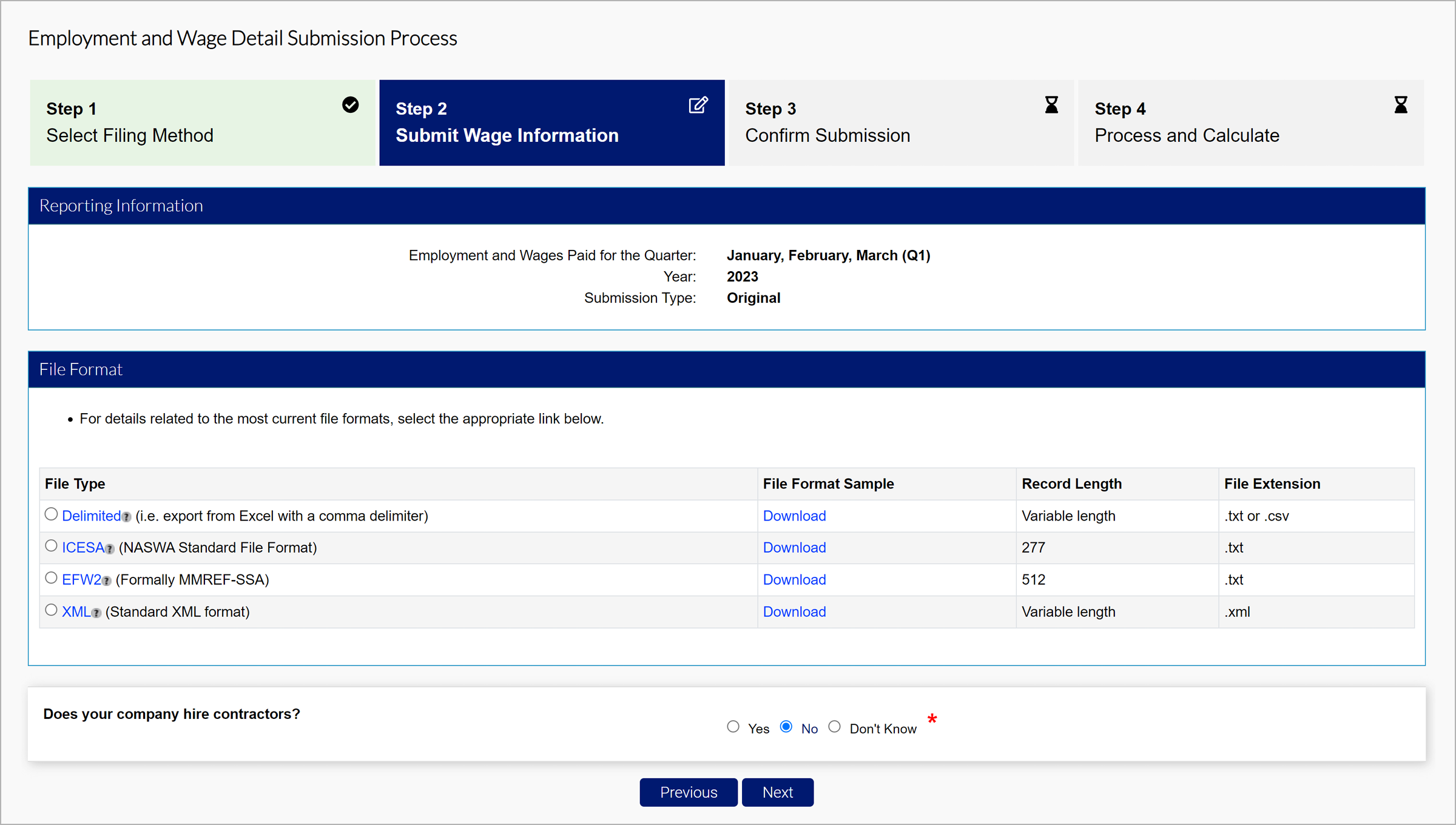The image is taken from a website detailing the "Employment and Wage Detail Submission Process." The image is divided into several sections, each representing a different step in the process.

1. **Step One: Select Filing Method**
   - **Visuals**: A light greenish-gray box with a white checkmark in a black circle located in the upper right-hand corner.
   
2. **Step Two: Submit Wage Information**
   - **Visuals**: A navy-colored box featuring a pencil on paper icon in the upper right-hand corner.
   
3. **Step Three: Confirm Submission**
   - **Visuals**: A gray box with an hourglass icon in the top right corner.
   
4. **Step Four: Process and Calculate**
   - **Visuals**: Another gray box, also with an hourglass icon in the top right corner.
   
Following these steps, there's a navy rectangle labeled "Reporting Information" in white font. 

- **Details**: 
   - "Employment and Wages Paid for the Quarter" section, specifying the months January, February, and March for Q1 of the year 2023.
   - **Submission Type**: Original.
   
Further down:
- **File Format**: Contains one bullet point.
- **File Type**: Features four clickable circles for selection.

The image is a comprehensive guide for users on how to submit employment and wage details for Q1 2023.